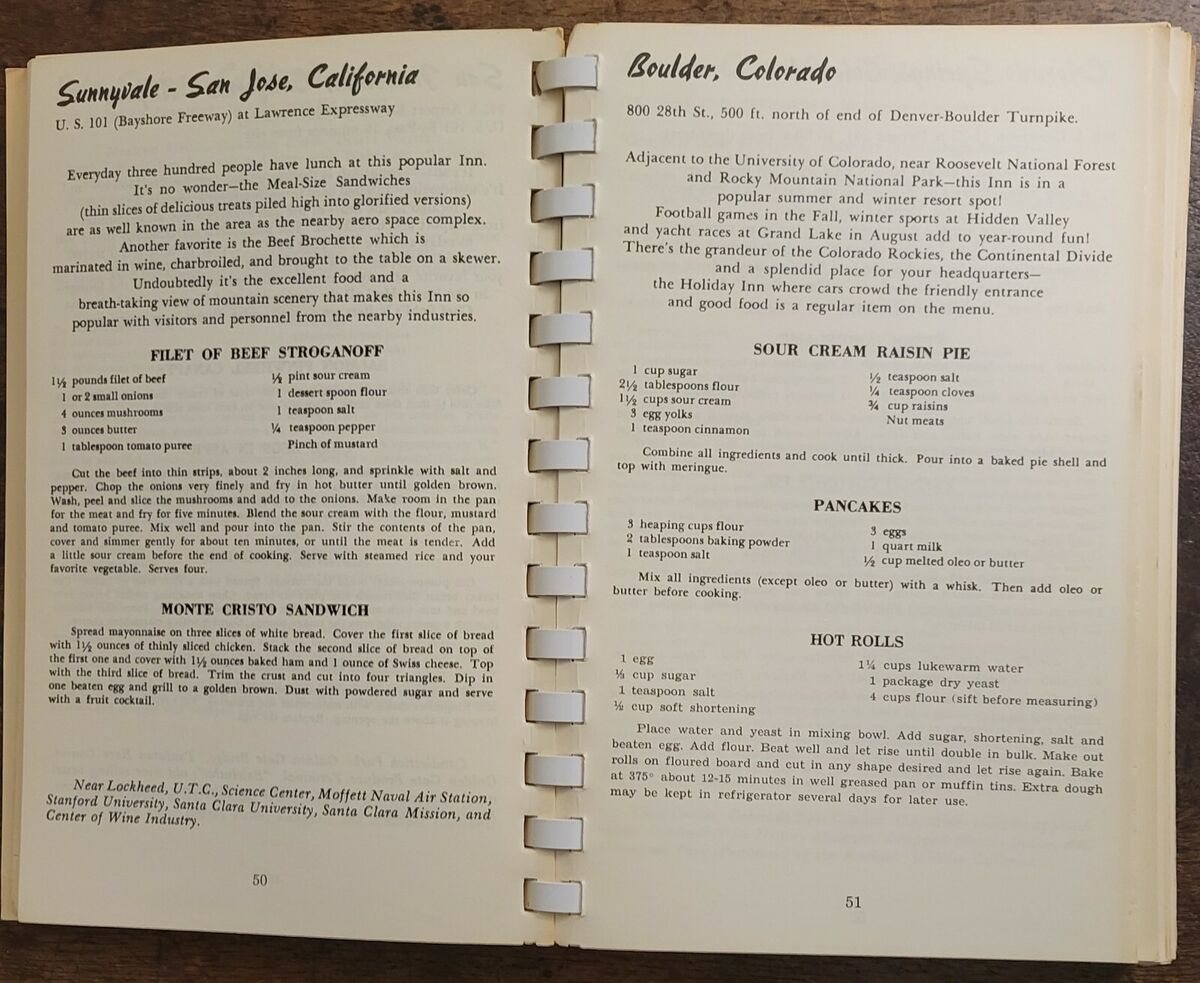The image depicts two open pages from a cookbook, placed on a brown wooden table. The book's binding runs vertically down the center, dividing the pages. On the left page, there are recipes associated with Sunnyvale, San Jose, California, including Fillet of Beef Stroganoff and Monte Cristo Sandwich. This section also mentions a popular inn on Lawrence Expressway known for its large meal-sized sandwiches and beef brochette, marinated in wine and charbroiled. The text highlights that this inn is frequented by 300 people daily, partly due to its excellent food and breathtaking mountain scenery. 

The right page features recipes from Boulder, Colorado, such as Sour Cream Raisin Pie, Pancakes, and Hot Rolls. The page details that these recipes are from an inn located at 828th Street, near the University of Colorado, Roosevelt National Forest, and Rocky Mountain National Park. This inn is noted for its popularity during summer and winter resort seasons, especially attracting crowds during fall football games. The setting includes sections of wood grain visible at the top and bottom of the image, emphasizing that the cookbook is resting on a wooden table. The colors in the image include white and black text on the pages, contrasted with the brown wood of the table.